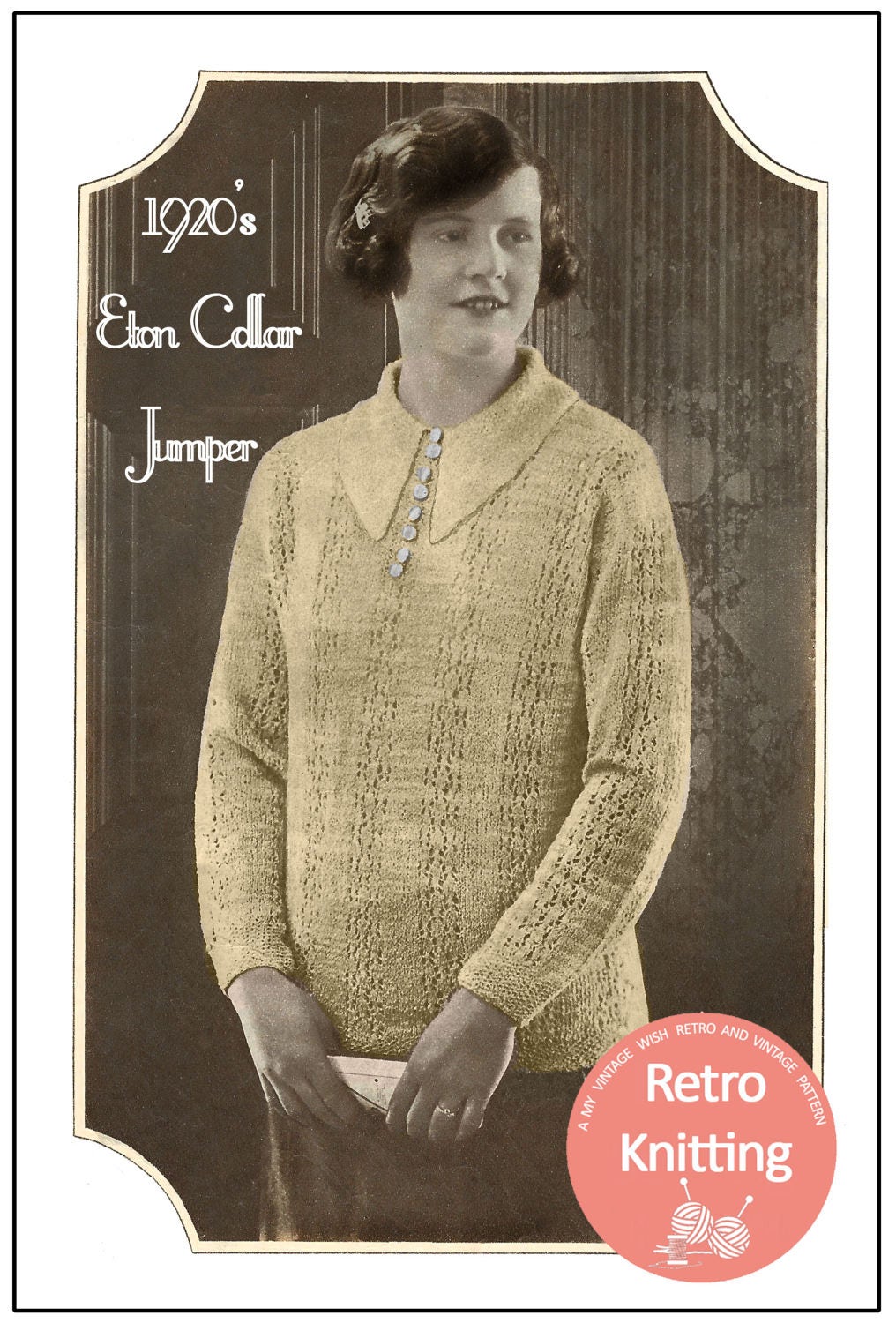This image is a vintage-style advertisement for a 1920s Eaton Collar Jumper. The sepia-toned photograph features a young woman with short brown hair that falls to her ears. She is half-smiling and looking off to her left, dressed in a yellowish-beige, full-sleeved, buttoned cardigan with a prominent Eaton collar, and paired with a brown skirt. The woman is holding some paper in her hands, and a ring adorns her left index finger. 

The background of the image is dark, enclosed by a white-bordered field and a black frame border. The advertisement's text is displayed in white, with "1920s Eaton Collar Jumper" positioned in the top left corner. The bottom right corner features a reddish-orange circular emblem with white text that reads "A My Vintage Wish Retro and Vintage Pattern" and "Retro Knitting," accompanied by illustrations of yarn balls with knitting needles.